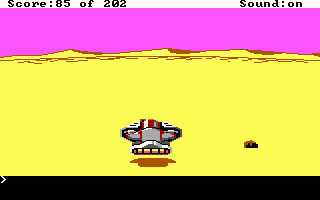The screenshot depicts a vintage-style video game reminiscent of classic DOS games but featuring more vibrant colors. Dominating the scene is a magenta pink sky that transitions into a vast, featureless white desert, punctuated by subtle yellowish sand dunes, hills, or cliffs seen in the background. In the center, a small, sleek spacecraft hovers above the desert surface, casting a shadow beneath it. The spacecraft is primarily white or gray with red accents and touches of yellow and orange near its exhaust, indicating some propulsion. In the lower portion of the screen, a black bar runs horizontally, featuring a less-than symbol (<) pointing towards the right, suggesting space for additional text. The upper-left corner displays the score: "85 of 202," while the upper-right corner indicates "sound: on."